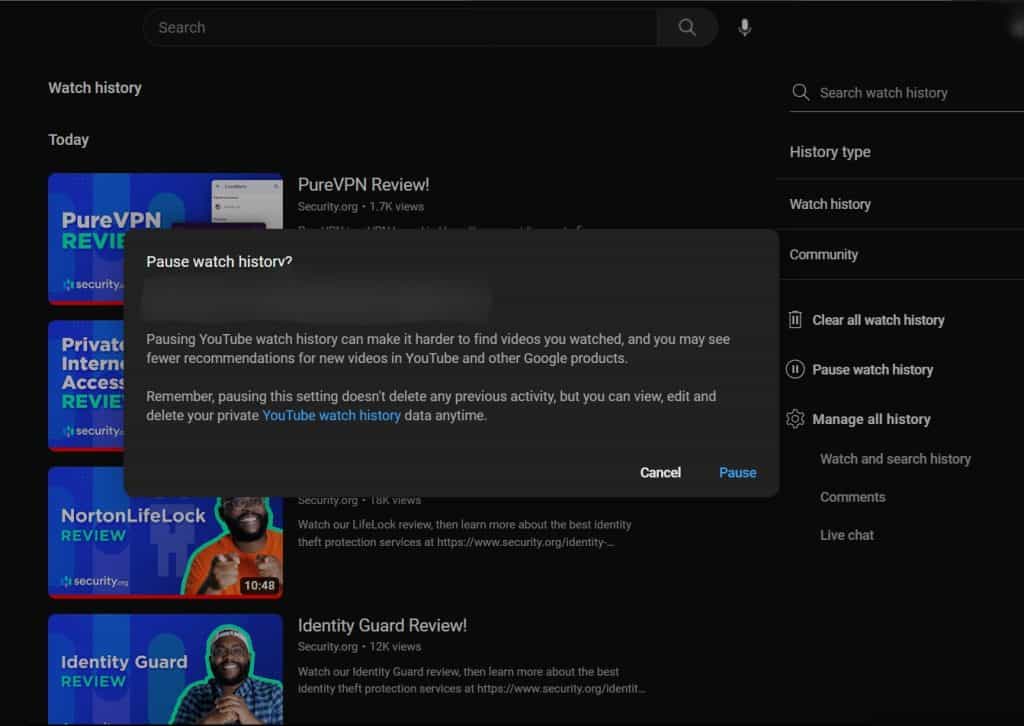A screenshot of YouTube's watch history page is depicted, captured in a landscape-oriented rectangle with a predominantly dark gray background. On the right side of the image, there is a vertical column with white text headings and options. The column begins with a search bar labeled "Search watch history," followed by headers for "History type," "Watch history," "Community," and other menu options. Additional features listed include "Clear all watch history," "Pause watch history," "Manage all history," "Watch and search history," "Comments," and "Live chat."

On the left side of the image, several previously viewed videos are displayed, each accompanied by blue thumbnails featuring white text and the green word "review" below them. The video titles include "Pure VPN Review" and "Identity Guard Review."

Overlaid on top of the page is a semi-transparent rectangular box with slightly rounded corners. This overlay contains white text at the top that reads "Pause watch history." Below this, redacted sections—obscured with a gray marker tool—presumably cover personal information. The overlay also includes a message explaining the consequences of pausing YouTube watch history:

"Pausing YouTube watch history can make it harder to find videos you watch and you may see fewer recommendations for new videos in YouTube and other Google products. Remember, pausing this setting doesn't delete any previous activity, but you can view, edit, and delete your private YouTube watch history data anytime."

At the bottom right of this overlay, two clickable options are available: "Cancel" in gray and "Pause" in blue.